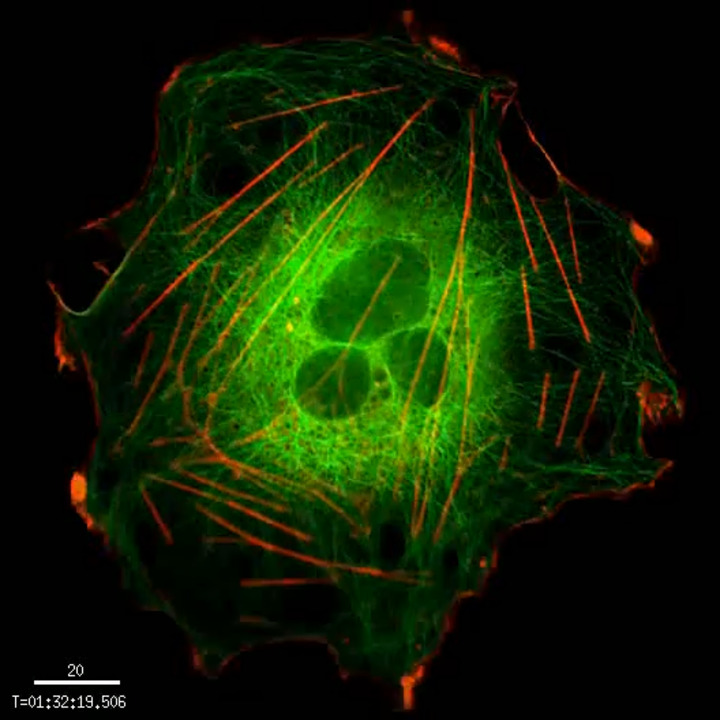In the center of the image, there is a close-up depiction of what appears to be a virus or molecule, primarily green in color. This central structure is somewhat round but not perfectly spherical, featuring ripples and an irregular shape. Within the main green area, there are three smaller green spheres, each emanating a bright green aura. Surrounding this core structure is a darker green, misshapen circular border with peculiar red lines resembling laser beams penetrating through it. The background of the image is entirely black, creating a stark contrast against the green and red elements.

Towards the bottom left of the image, there is a legend displaying the number "20," followed by a thick white line. Below this line, there is a numerical timestamp reading "T = 01:32:19.506," likely corresponding to a specific moment in an ongoing scientific observation or experiment. The image has a highly scientific appearance, possibly inspired by microscopy or molecular visualization techniques.